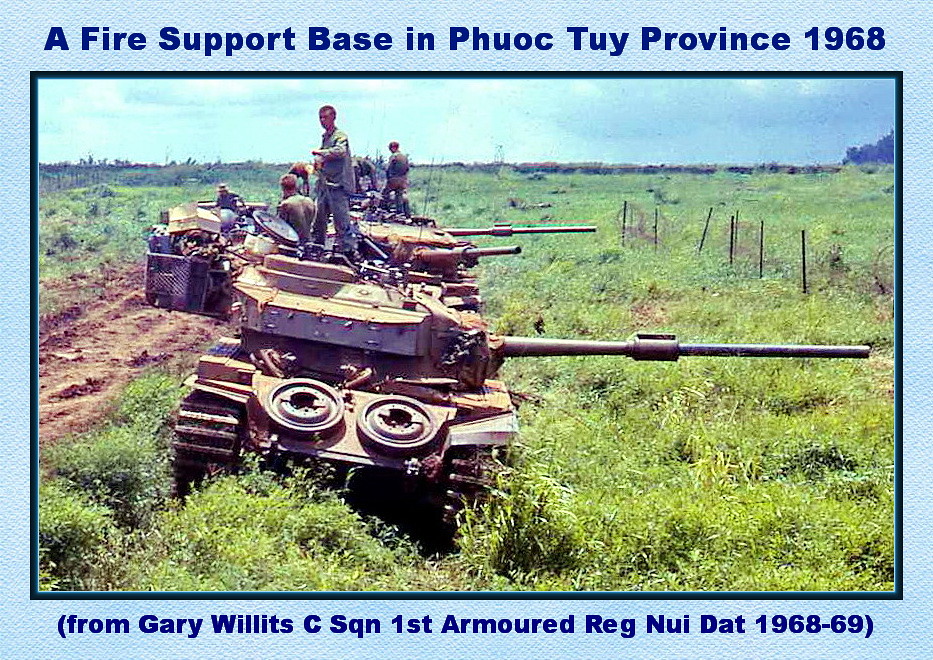The image resembles a postcard with a light blue background and a dark blue border surrounding a central photograph. In bold blue capital letters at the top, it reads: "A FIRE SUPPORT BASE IN PHUOC TUY PROVINCE 1968." Below the photograph, the text in capital and lowercase letters states: "FROM GARY WILLETT C-SQUADRON, FIRST ARMOURED REG NUI DAT 1968-69." The photograph itself depicts a row of tanks in a field, their gun barrels pointing towards the right side of the image. On top of the tanks, men dressed in green fatigues are standing. In the background, one can see a fence and a blue sky, enhancing the scene's expansive feel. Detailing on the tanks includes open lids and storage bins.